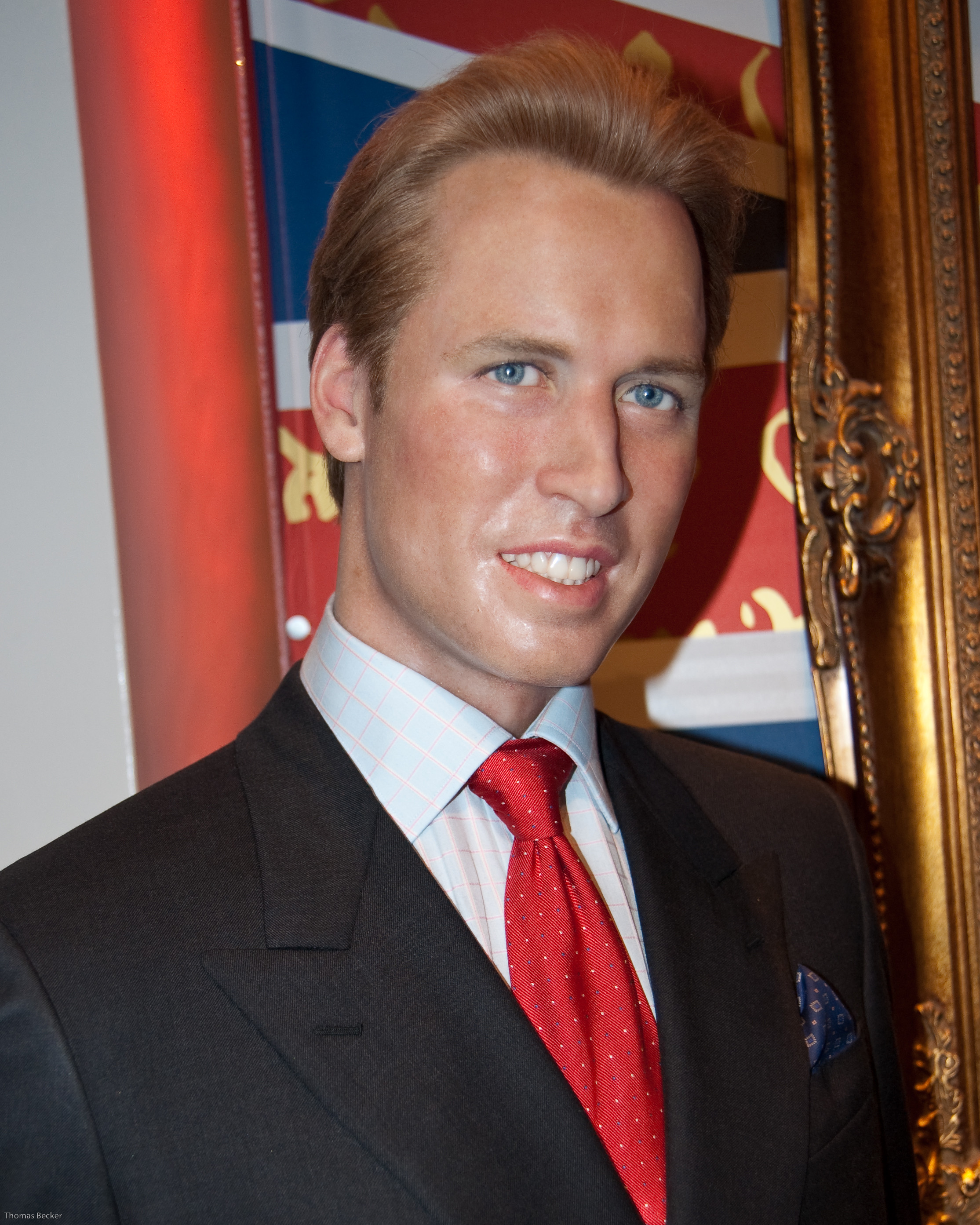The image captures a handsome man, likely in his late 20s to early 30s, with dark blonde hair neatly combed back. His blue eyes and broad smile reveal his bright white teeth. He is dressed in a dark charcoal suit, paired with a white dress shirt and a red tie adorned with small, white polka dots, tied in a Windsor knot. Adding a sophisticated touch, he has a blue pocket square peeking from his suit jacket. The background shows him standing indoors, against white walls with a red and blue color block. To his left, there is an intricate, gold-framed picture with a reddish hue, possibly depicting a flag. The man is slightly turned to his left, allowing only one ear to be visible.